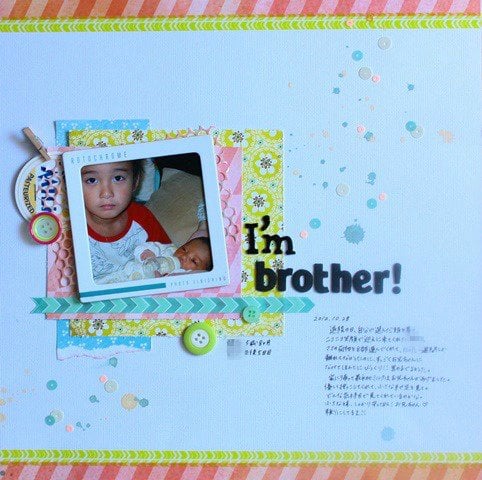The image depicts a heartfelt celebration of siblinghood, featuring a young boy proudly holding his newborn brother. Both children are prominent in the picture; the older brother wears a red and white striped shirt, while the baby is dressed in a white onesie and has a bottle in his mouth. The baby's complexion suggests a possible Hispanic heritage. The setting appears to be a cozy home environment, with the siblings sitting on a bed.

The photo is part of a creatively decorated flyer or craft project. It is bordered on the top and bottom with a candy cane-like pattern of red and pink diagonal stripes, and just above those stripes are thin yellow lines. The central background is predominantly blue, adorned with playful circles and splashes of various shades of blue. Additional decorative elements include green and red buttons and a yellow flower and pink-patterned frame. Text on the right side of the image reads "I'M BROTHER!" in bold black letters, alongside a handwritten date, "10-28-2013," and some text in an Asian language, likely Chinese. The flyer projects a vibrant and joyful atmosphere, capturing a precious family moment.